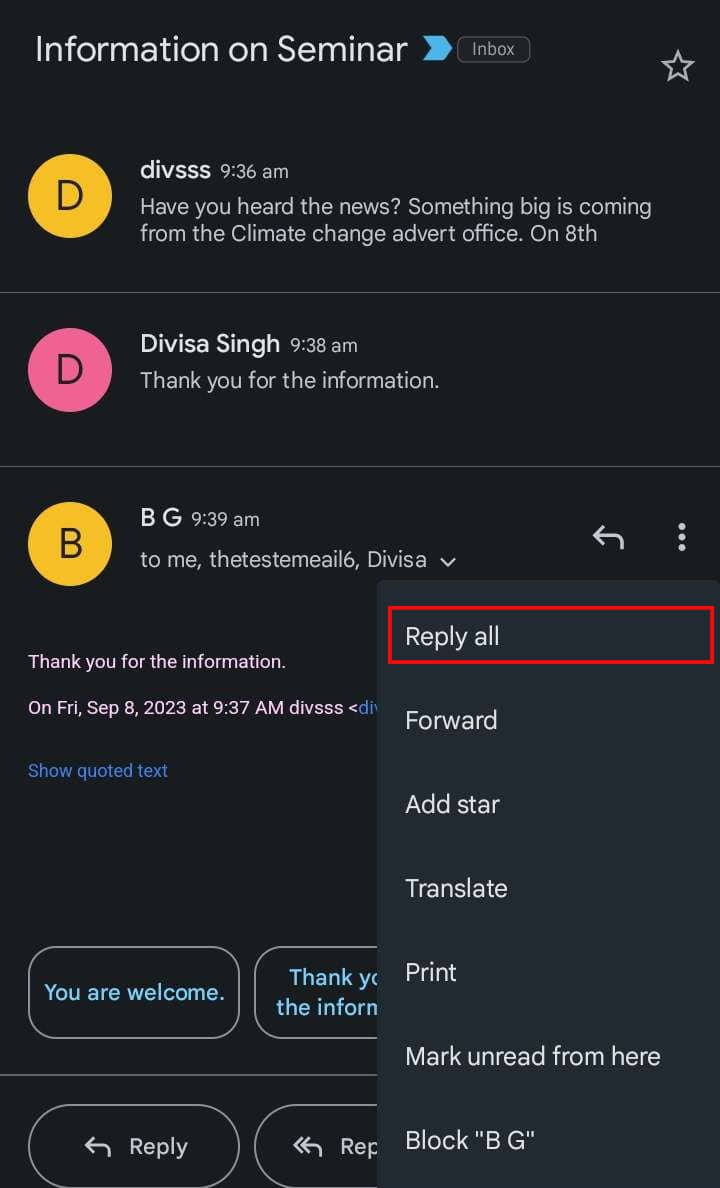**Descriptive Caption:**

Against a black background, the image features the text "Information on Seminar" in white at the top. Below this, a blue arrow leads to the word "Inbox," with a white star icon positioned on the right side. The content is divided into three distinct sections:

1. **First Section:**
   - A yellow circle with the letter "D" inside.
   - Accompanying text reads: "Diviss, D-I-V-S-S-S. Have you heard the news? Something big is coming from the Climate Change Advert Office on 8th."

2. **Second Section:**
   - A pink circle with a capital "D" inside.
   - The text says: "Divissing, capital D-I-V-I-S-S-A, capital S-I-N-G-H. Thank you for the information."

3. **Third Section:**
   - A yellow circle with the letter "B" inside, followed by the initials "B.G." in white.
   - The text reads: "To me, Divissing. T-H-E-T-E-S-T-E-M-E-A-I-L, number six, comma, capital D-I-V-I-S-A. Thank you for the information. Show quoted text."

At the bottom of the text, options such as "Reply all," "Forward," "Add star," "Translate," "Print," "Mark unread from here," and "Block B.G." are listed, with "Reply all" highlighted by a red outline.